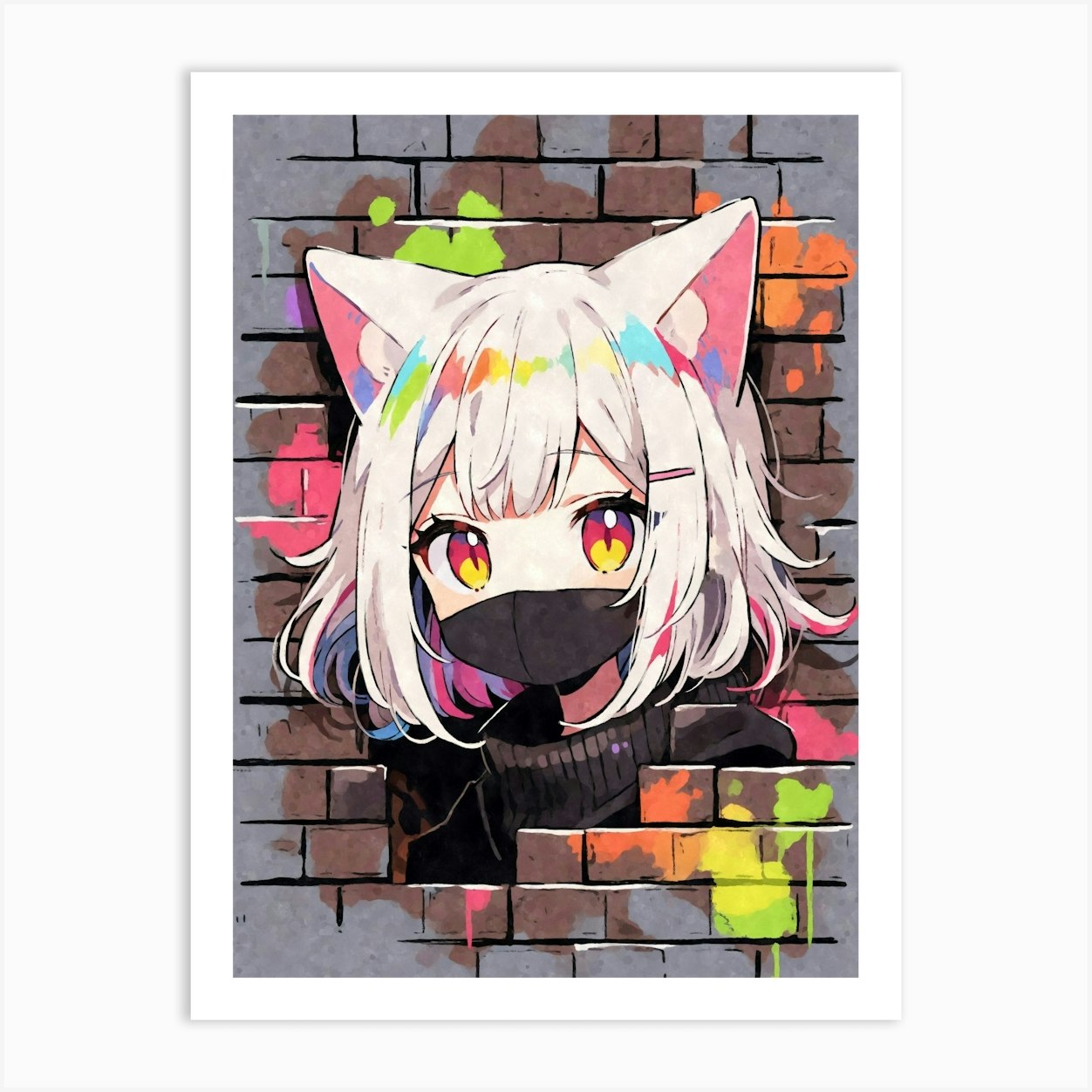The image shows a digital artwork mounted on a grey-colored wall. The painting itself features a grey brick-patterned background with splashes of vibrant colors including green, orange, pink, yellow, brown, and purple scattered throughout. At the center of the artwork is an anime girl’s portrait, focusing on her head, neck, and the upper part of her shoulders. The girl has short white hair styled in French curls and adorned with large, triangular ears that are pink and white at the tips. Her eyes are large and multicolored, with hues of yellow, blue, and pink, framed by black eyelashes. She wears a grey hygiene mask that covers her nose and mouth, and a grey turtleneck shirt. The mask and shirt blend seamlessly into the brick-patterned background, giving the illusion that she is emerging from the wall. The bottom right section of the painting showcases splotches of green, yellow, orange, and pink, while the top right features orange, and the left side has green, purple, and pink colors. Additionally, her bangs are streaked with multicolored highlights, adding to the overall vibrancy of the piece.